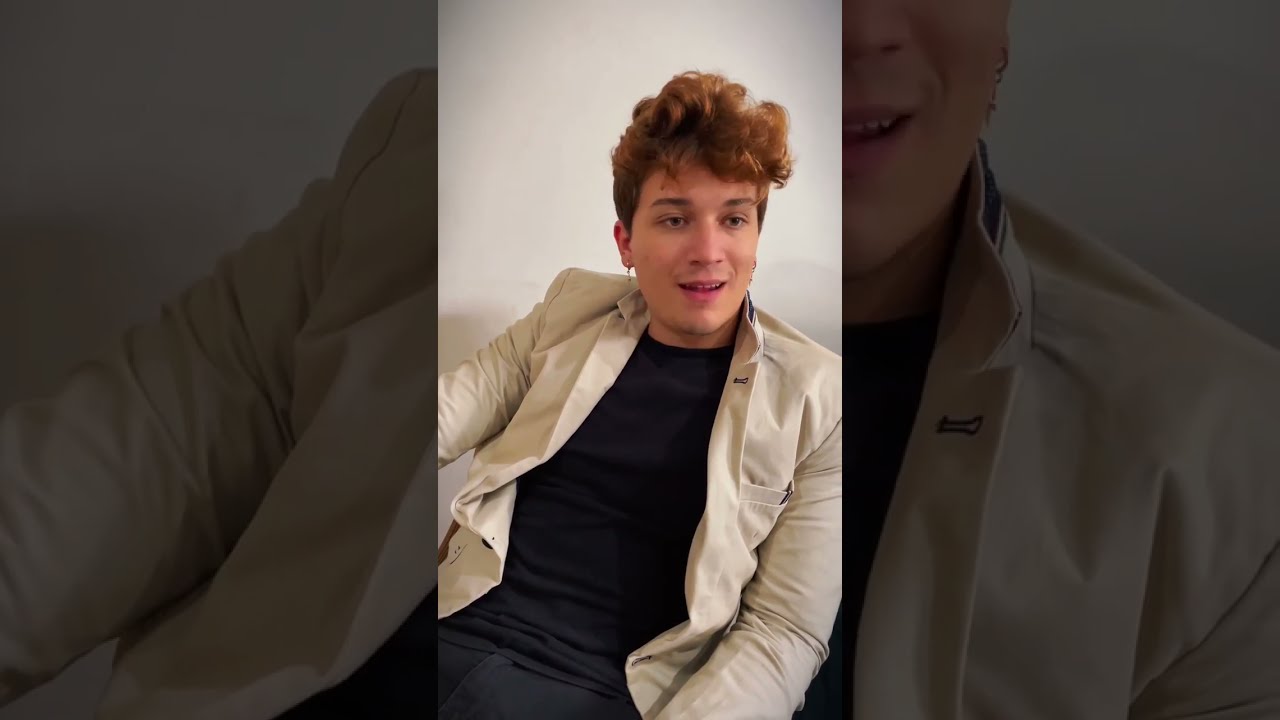In the image, we see a young man of Caucasian descent, sitting in a room with a white and gray background. He appears to be looking off to the left, possibly in mid-conversation, with a slight smile on his face. He's dressed in an open, long-sleeved beige jacket over a black shirt, paired with black jeans. His distinctive hairstyle features thick, curly, reddish-brown hair on top, cut short on the sides. He sports a faint mustache and some chin whiskers. Adding to his look, he has pierced ears adorned with dangly earrings and a hint of lip gloss. 

The image itself has been creatively edited: a darkened, enlarged version of the photo serves as a backdrop for the central, original photo of him.